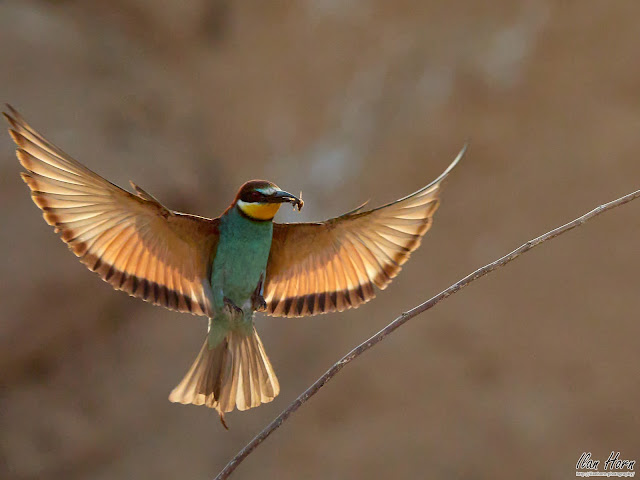The photograph, likely taken outside, showcases a bird caught mid-flight, set against a blurred, brown-hued background indicative of a forest in fall. Dominating the center right of the image is a bare twig that rises diagonally from the bottom left towards the center right, continuing off-screen. The bird, depicted in sharp detail, hovers just to the left of this twig, its wings fully outstretched without motion blur. The bird's head is brown, with a distinct white area just above its thin, curved black beak. Below the beak, a bright yellow patch transitions into a white edge, followed by a contrasting black band around the neck. Its body is a striking seafoam green, while the wings are tan, with darker brown tips. The tail feathers are similarly light brown. In the bird's beak, a small bug or bee is visible. In the lower right corner of the image, the text "Elon Horn" appears in black against a white outline.